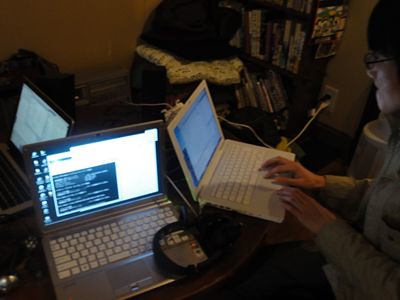This photograph features a setting with three open laptops on a dark brown table, indicating a shared workspace. In the right forefront, a woman with dark hair, wearing glasses and a long-sleeve jacket, is actively working on a white laptop. Her face, partly visible, is cast in shadow, showing concentration as her hands rest on the keyboard. To her left, closer to the photographer, is a silver laptop facing the camera, with a pair of headphones resting atop it. Behind these, a third laptop is visible, facing to the left. The background showcases a fully stocked bookshelf filled with small, thin books, and an additional chair suggesting more seating in the area. The walls are yellow, adding warmth to the room, and a cord extends from beside the bookshelf, disappearing out of frame. The overall scene gives an impression of a quiet, studious environment.